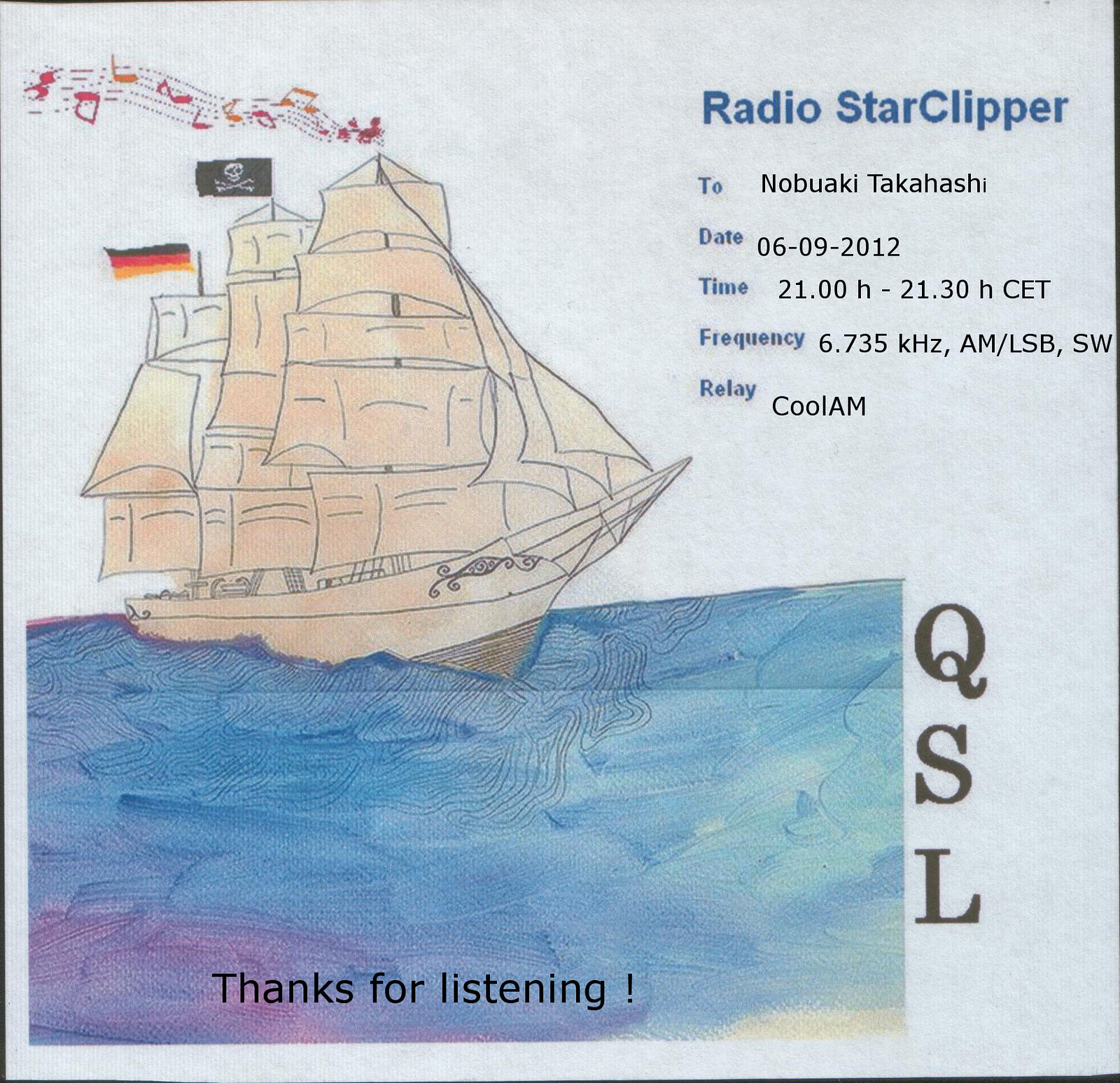This image displays a scanned flyer printed on light gray paper, predominantly featuring a detailed watercolor painting of a sailing ship on the ocean. The top of the flyer prominently showcases a logo of a skull and crossbones on a pirate flag, accompanied by another flag, possibly German, with black, red, and yellow stripes. Below the logo, a musical staff with notes in red and orange flies from the highest mast, adding a dynamic visual element. 

Centered on the flyer is a beautifully painted pirate ship with numerous sails, rendered with pencil lines and filled in with tan watercolor. The ship floats on a swirly depiction of the ocean painted in varying shades of blue, pink, and purple, complete with shadows and reflections to enhance depth. Music notes appear to be floating around the ship, adding an artistic touch to the nautical scene.

In the upper right section, bold blue text reads "Radio Star Clipper," and below it, the recipient’s name "Nobuaki Takahashi." Detailed information follows in a mix of blue and black text, listing the date (06-09-2012), time (2100 hours to 2130 hours CET), and frequency (6.735 kilohertz AM/LSB, SW) of the broadcast. The word "relay" is printed in blue followed by "cool AM" in black. In the lower right corner, the bold, capitalized letters "QSL" are printed. Nestled at the bottom of the sea illustration, the message "thanks for listening!" adds a warm thank-you note to the receiver.